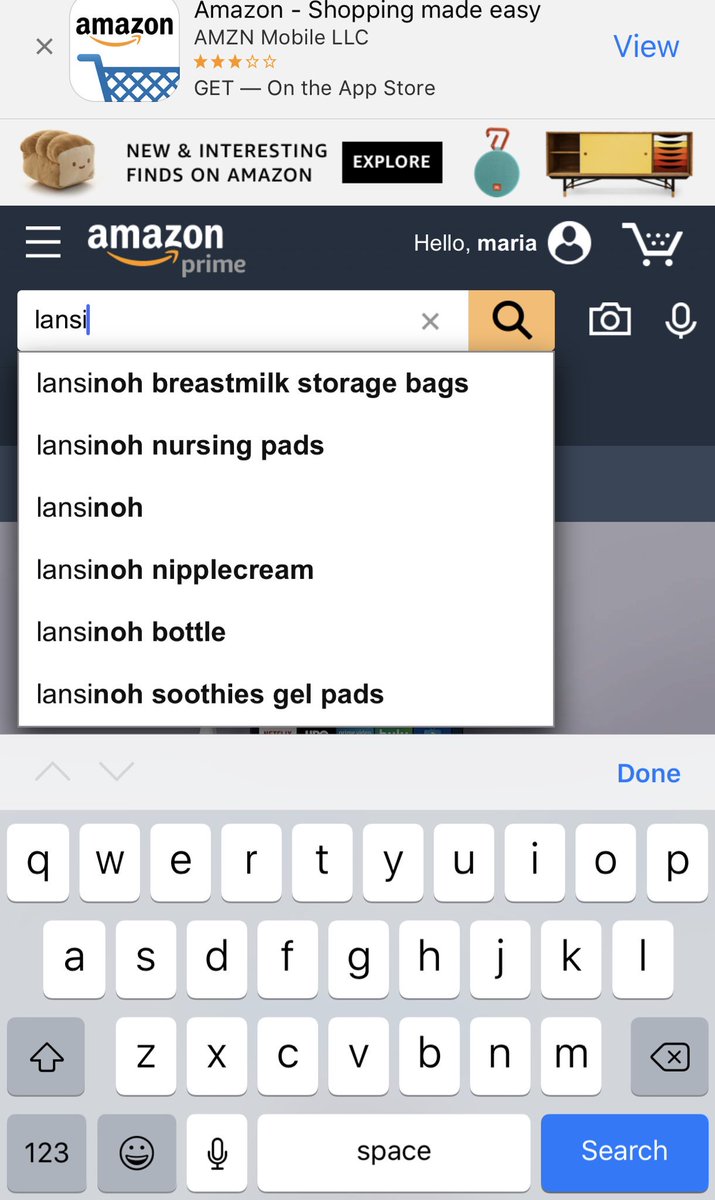This image captures a screenshot of the Amazon mobile website, likely viewed on a smartphone. The heading at the top features a gray section that reads "Amazon Shopping Made Easy" and mentions "Amazon Mobile LLC" with an option to "Get it on the App Store" in blue text on the right side. Just beneath, a section titled "New and Interesting Finds on Amazon" showcases various items including a stuffed animal resembling a loaf of bread next to a black "Explore" button, a round ball with red wires, and a TV console.

At the center of the screen, there is a promotional banner for Amazon Prime saying "Hello, Maria" next to a generic profile picture icon. Adjacent to this banner are icons for a shopping cart, a camera, and a microphone. Below, the search bar shows recent searches for "Lansinoh," and the results display items such as Lansinoh Breast Milk Storage Bags, Lansinoh Nursing Pads, Lansinoh Nipple Cream, Lansinoh Bottles, and Lansinoh Soothies Gel Pads. The bottom portion of the screen captures a digital keypad, indicating that this screenshot was taken on a mobile device.